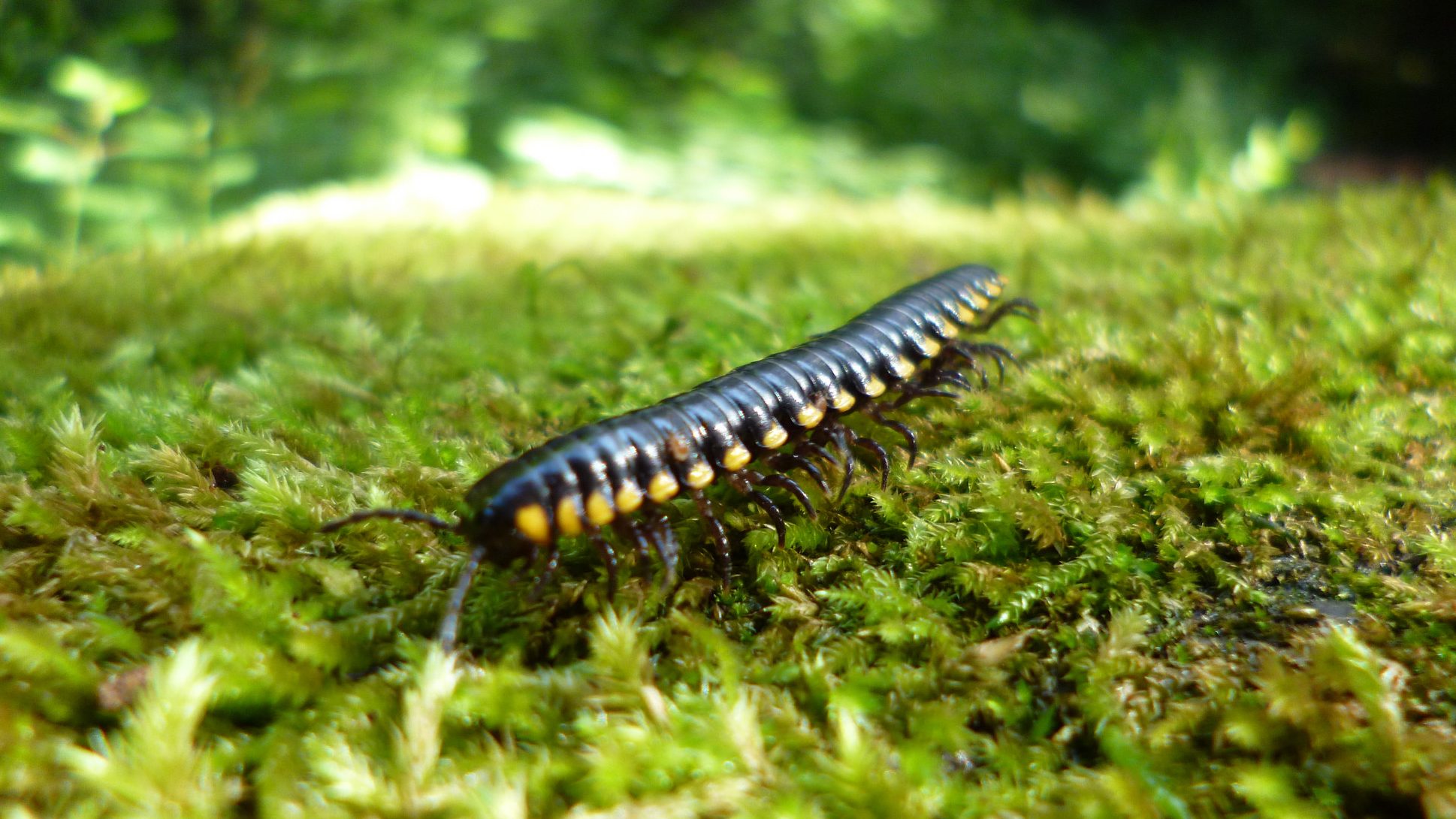This is a detailed, horizontally oriented color photograph set outdoors. It captures a realistic-looking scene of a long insect, most likely a centipede or millipede, crawling on a lush, green grass surface. The grass and perhaps other plants form an in-focus foreground, while the background is out-of-focus greenery, adding depth to the image. The insect, situated in the center of the frame, is predominantly black with numerous legs along its sides. It features distinctive yellow dots or circles running along its body, particularly near the legs. The creature appears to be a few inches long, with the length almost resembling that of a small snake. It has long black antennae situated towards the front, which is directed towards the bottom left corner of the photograph, while its tail extends towards the top right. The image is well-lit, highlighting the intricate details of the insect and the vibrant green surroundings.